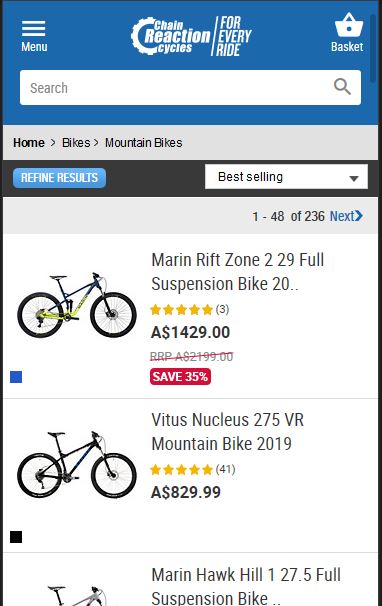This is a caption that somebody gave for an image using their voice. Clean it up and formulate it into a descriptive caption. Make it very detailed.

Here we have a screenshot of a website that is selling bicycles. The app appears to be being viewed on like a vertical style so it makes me think more phone or tablet or app than being viewed on like a desktop website or anything like that. In a blue border at the top there is a white three horizontal line icon that says menu. There is a logo up there with a kind of like a cogwheel style design that says chain reaction cycles with a slash mark after it that says for every ride. In the upper right hand corner there is a basket like a shopping basket style icon but it's not like a cart but like a basket you would carry for this particular style. Below is a white search bar with a gray colored magnifying glass for search. It says home bikes and mountain bikes as the kind of filtered there. It says refine results in the blue button below that with best selling as the picked option. 1 of 48 of 1 through 48 of 236 with the next button here and then you have a image of a bike in black and green and an image of a bike in black. The first one says Marin Rift 229 full suspension bike five-star review with three reviews a dollar sign for 1429.00 save 30% then a Vitus Nucleus 275 VR mountain bike 2019 41 five-star reviews a dollar sign 829.99

---

Descriptive Caption:

This image is a screenshot of a vertically-oriented mobile app displaying a website that sells bicycles. The top section has a blue border containing a white menu icon (three horizontal lines) labeled "Menu". Next to it is a logo designed like a cogwheel, displaying the text "Chain Reaction Cycles" followed by the slogan "For Every Ride". In the upper right corner, there is a shopping basket icon styled like a hand-carry basket.

Below the header, a white search bar with a gray magnifying glass icon is available for searching. The breadcrumb navigation shows the categories "Home", "Bikes", and "Mountain Bikes". There's a blue "Refine Results" button, and "Best Selling" is highlighted as the selected filter option.

The product list shows items 1 through 48 out of 236 on this page, with navigation buttons to move to the next set of results. Featured products include two bikes: 

1. A black and green "Marin Rift Zone 29" full suspension bike, rated with five stars based on three reviews, priced at $1,429.00 with a 30% discount.
2. A black 2019 "Vitus Nucleus 275 VR" mountain bike with 41 five-star reviews, priced at $829.99.